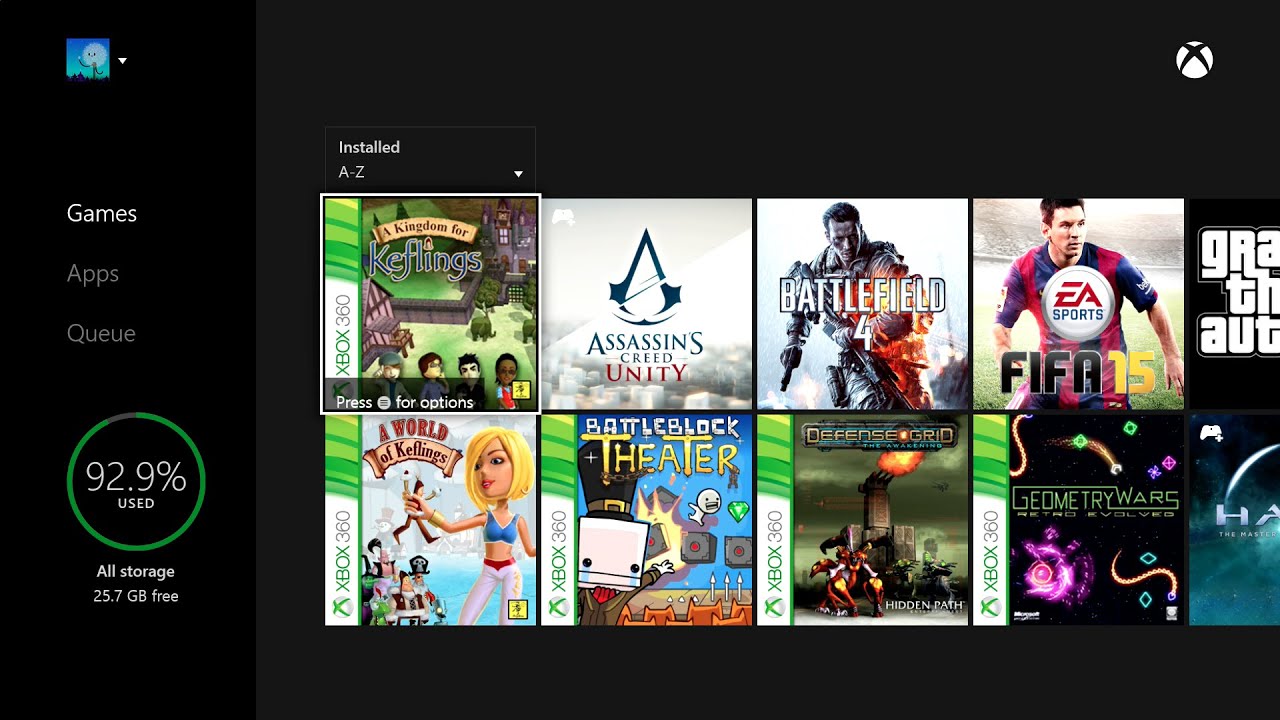A detailed screenshot of an Xbox user interface displaying the owner's profile and game library. The predominant feature is a black background with the unmistakable Xbox logo. The interface showcases a variety of game cover images, albeit the titles are difficult to distinguish. Recognizable game icons include prominent ones like FIFA, Battlefield, and Grand Theft Auto, suggesting the user's diverse gaming interests. The storage usage indicator reveals the user has utilized 92.9% of their available storage, emphasizing their extensive engagement with gaming. The colorful game thumbnails stand out against the otherwise minimalist black background, adding vibrancy to the interface.